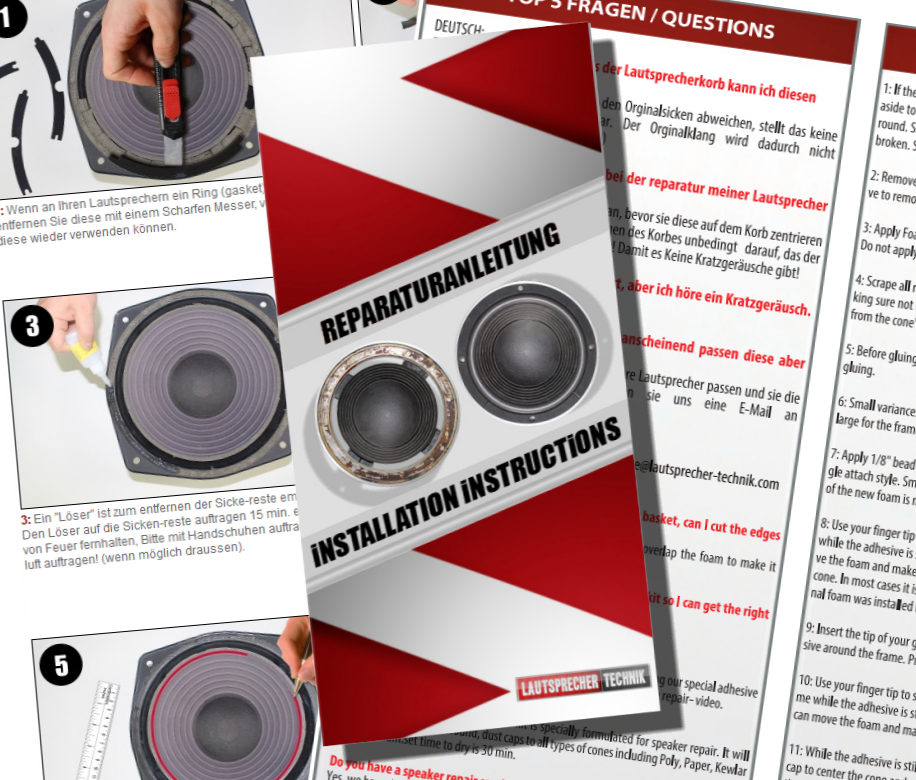The image is a close-up of a detailed installation instruction sheet for a car phone speaker, presented in full color. The square image features multiple smaller, numbered diagrams (at least 1, 3, and 5) laid out without a border or specific background. 

In the top left corner, there's a round black spot with the number 1, showing a photograph of someone's hand using a retractable blade on the speaker. Directly below, labeled number 3, another photograph depicts a Caucasian hand applying glue to the speaker. At position number 5, the same hand is shown applying glue to the upper right corner of the speaker. 

A distinguishable part of the image is a gray speaker with concentric lines that get smaller towards the center. An essential element of the instruction is marking the speaker with a red line, shown in one of the steps.

Additionally, there is a pamphlet featuring red and white markings with German text. The open pamphlet has visible instructional text, including a section that starts with the letter 'R' and mentions installation instructions. A part of the pamphlet is in Dutch, with some English instructions largely cut off, including an area titled "Questions" addressing common inquiries about the installation.

The clear, comprehensive visuals and multi-language text emphasize step-by-step speaker installation, distinguishing between old and new speaker components within the instructional guide.